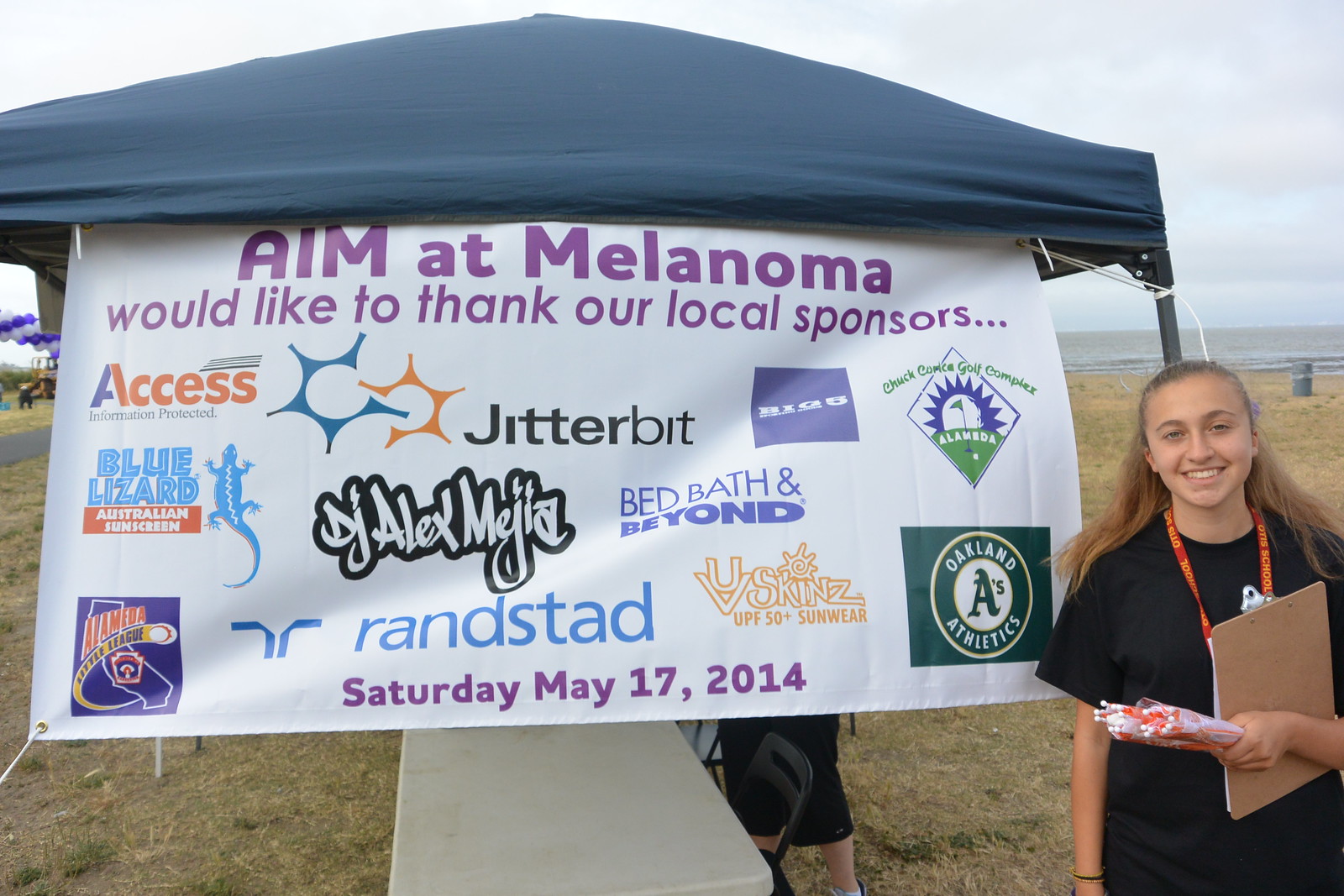In this wide rectangular outdoor image, a woman stands on the far right in front of the edge of a tent, which is supported by gray poles. The tent’s bluish-gray canvas roof extends across the image and curves slightly upward towards the center. A white rectangular sign hangs underneath the tent, reading "AIM at Melanoma would like to thank our local sponsors" in purple font. Below this heading are various company logos, including recognizable names like Oakland A's, Jitterbit, and Bed Bath & Beyond, with the date "Saturday, May 17th, 2014" also in purple at the bottom. The scene is set in a large, flattened grassy field that appears brownish-green, with subtle hints of water and clouds in the background suggesting a possible oceanic proximity. The woman, dressed in a black t-shirt, holds a clipboard and an orange ribbon, which might be a pass, while smiling directly at the camera. A partial white table and an indistinct leg are visible behind the banner under the tent, contributing to the bustling yet inviting atmosphere of this event.